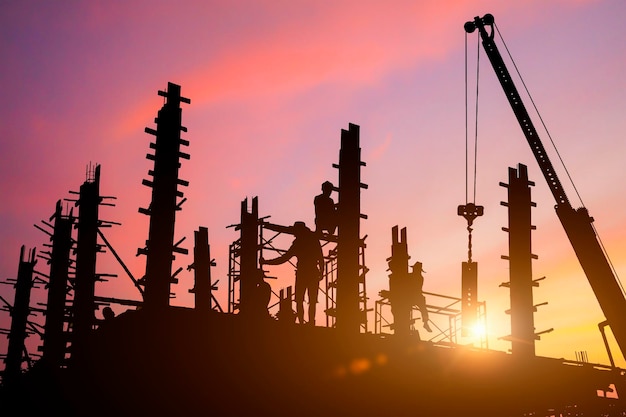In this captivating image, the scene is set at either dawn or dusk, evidenced by the vibrant sky painted in hues of purple, pink, and orange, with a touch of blue. The sun, either rising or setting, sits just above or behind the skeletal frame of a high-rise building under construction. The entire foreground, including the structure, a crane to the right, and the figures atop the building, is rendered in stark black silhouette, creating dramatic contrast against the colorful sky. The crane extends into the sky, though only its top part is visible, adding further to the industrial atmosphere. At least five workers can be discerned, their outlines suggesting various postures, from standing to sitting. One figure, perhaps a child, is kneeling on the structure. This silhouetted tableau of human activity on the unfinished edifice offers a striking study of form and shade, capturing the essence of early or late hours on a construction site.